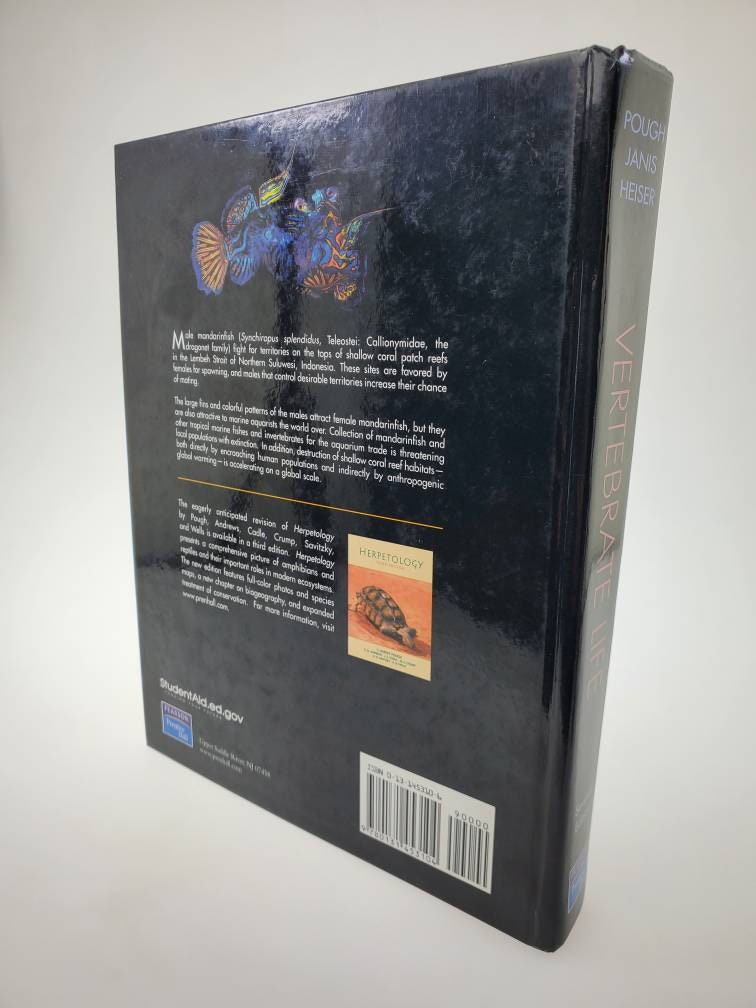The image showcases the back cover of a black book, viewed at an angle against a light gray, almost white background. The book stands upright, exposing the spine partially. The spine text at the top in blue reads "Pau Janis Heizer," and in red further down, it says "Vertebrate Life." The back cover features a colorful drawing at the top, depicting a fish with a blue body and orange fins. Below the drawing are three paragraphs of white text, with a thin yellow stripe separating the second and third paragraphs. Adjacent to the third paragraph, on the bottom right, there's a barcode, and next to it is an image of another book cover, which is tan-colored, titled "Herpetology" with a green font, and it has a depiction of a turtle. Additionally, the left lower corner includes the text "studentaid.ed.gov".